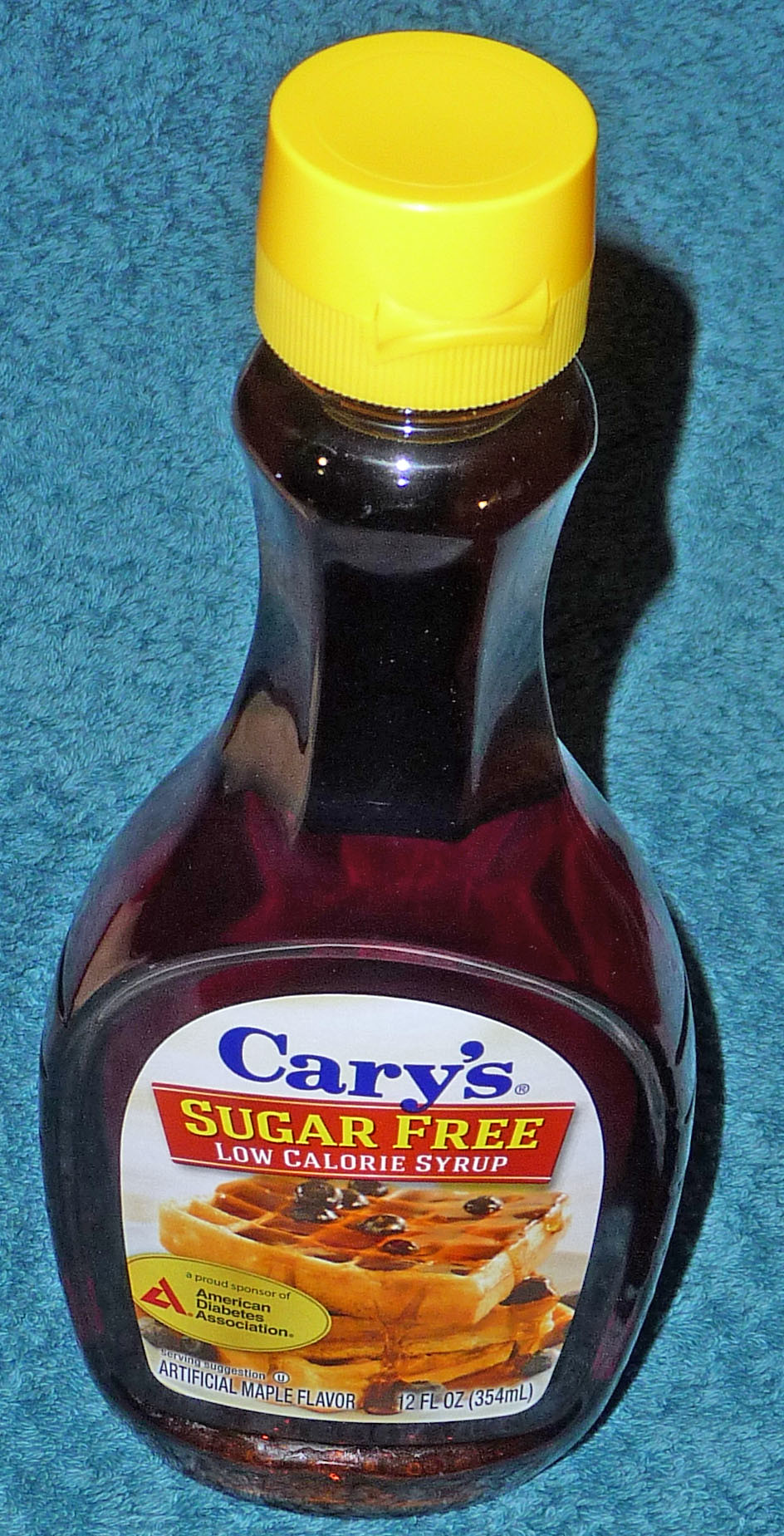This image depicts a bottle of Cary's Sugar-Free Low-Calorie Syrup from a top-down perspective, resting on a marbleized light blue and darker blue counter. The bottle is equipped with a yellow pop-open cap, and the syrup inside is a rich golden brown. The bottle's white label prominently displays "CARY'S" in blue lettering, accompanied by a red rectangle featuring "SUGAR FREE" in yellow and "LOW CALORIE SYRUP" in white. Below the text, there's an image of waffles topped with blueberries, drenched in syrup. Adjacent to the waffle image, a yellow oval highlights the product as "a proud sponsor of the American Diabetes Association." At the bottom of the label, in blue text, the description reads "ARTIFICIAL MAPLE FLAVOR, 12 fluid ounces, 354 milliliters."